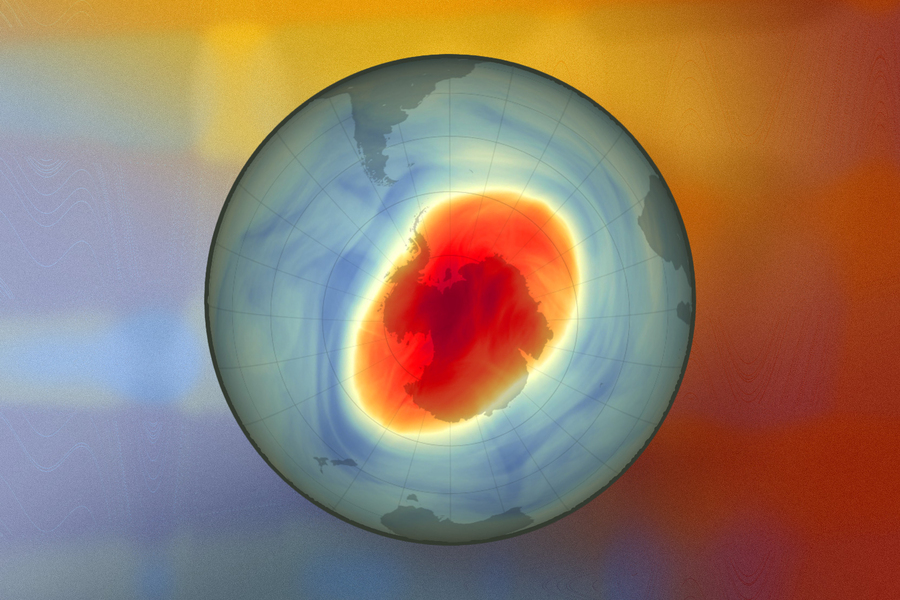This image features a vibrant, circular design reminiscent of a geographical representation. Dominating the center of the circle is a prominent oval-shaped object. This oval is outlined in a striking white-yellow hue and filled with a vivid orange color. Nestled within the orange oval is a smaller shape that resembles the outline of a state. Surrounding the central oval, the circular space is adorned with varying shades of blue, transitioning from a lighter blue to a darker blue towards the edges. Interspersed within the blues are subtle touches of gray, contributing to the overall composition. The entire image evokes the sensation of gazing down at a globe from above, capturing the intricate detail and complex beauty of our world's terrain.